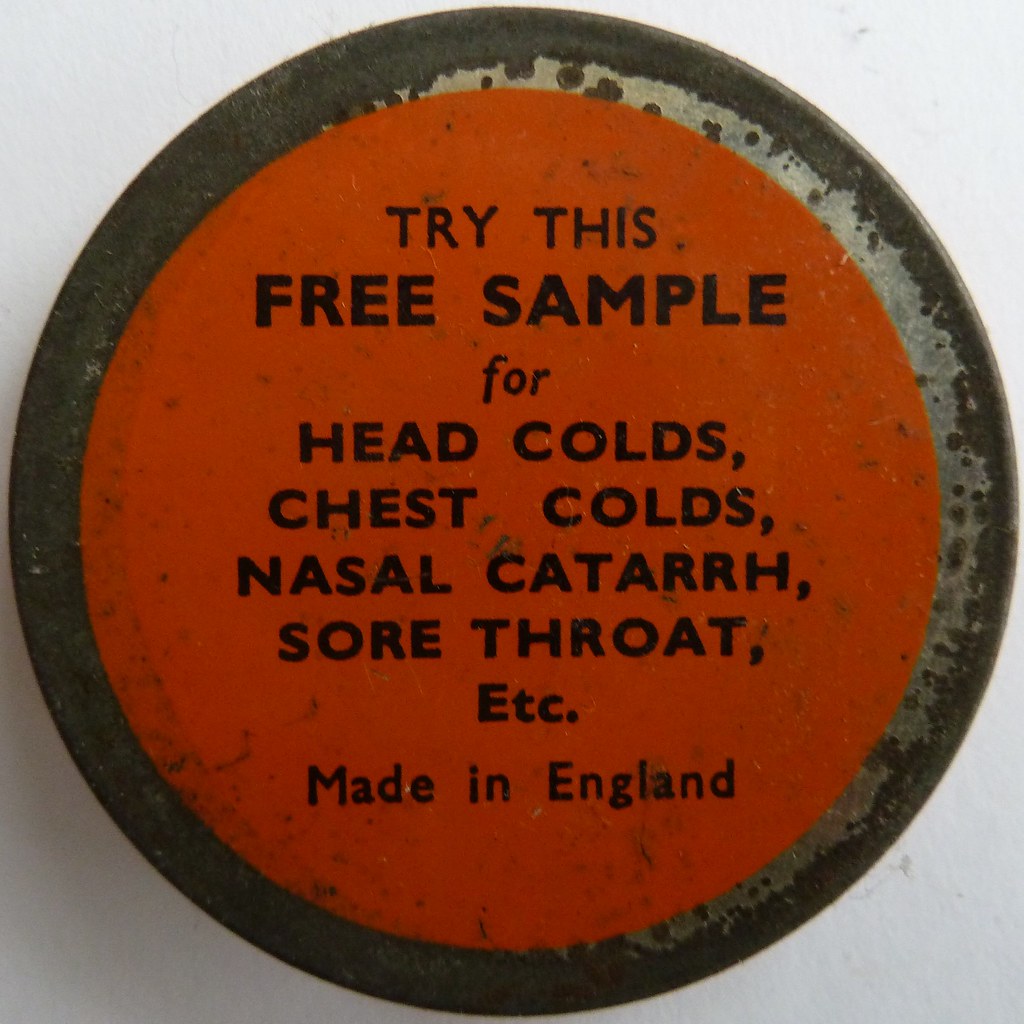The image depicts a close-up of the top of an old, circular metal tin, likely a free sample of a medicinal product. The tin's lid is notably corroded and rusted, with visible wear along the edges. An orange sticker, or possibly paint, covers the top, displaying black text that reads, "Try this free sample for head colds, chest colds, nasal catarrh, sore throat, etc. Made in England." This strongly suggests it is an antique medication, probably from the late 1800s or early 1900s. The black letters on the sticker are slightly chipped, adding to the aged appearance of the tin. The tin is positioned on a white or beige surface, which is only visible in the corners of the photo.